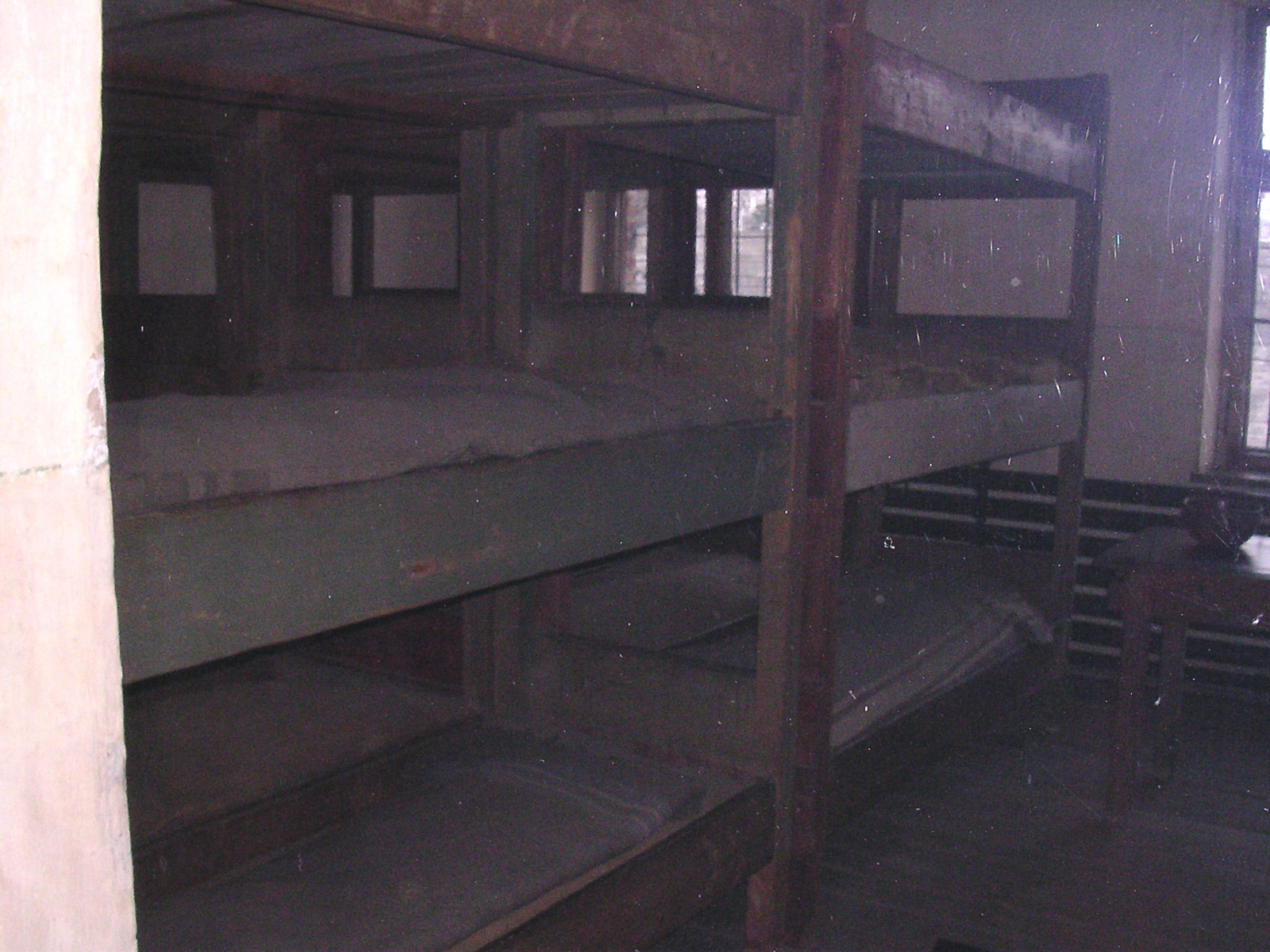The photograph displays a dark, aged room, possibly in an old camp cabin or even reminiscent of a historical setting like a concentration camp, characterized by its worn and weathered elements. The focus is on a set of three-tiered bunk beds made from old, chipped, and fading wooden frames, some of which show remnants of olive green and beige paint. The beds are sparsely furnished with thin mattresses and possibly some blankets. The room appears to have been captured from the doorway, enhancing the sense of desolation. To the right side of the bunk beds stands a dark brown, square nightstand with an indistinguishable bowl atop it. The walls are a mix of faded beige, white, and spots where the paint has worn to reveal pink and light brown hues underneath. They show signs of significant aging and deterioration. In the background, several windows lined with wood allow a faint light to filter in, hinting that it is daytime. Below these windows are wooden railings. The floor appears to be made of dark hardwood, adding to the somber and antiquated atmosphere of the photograph.